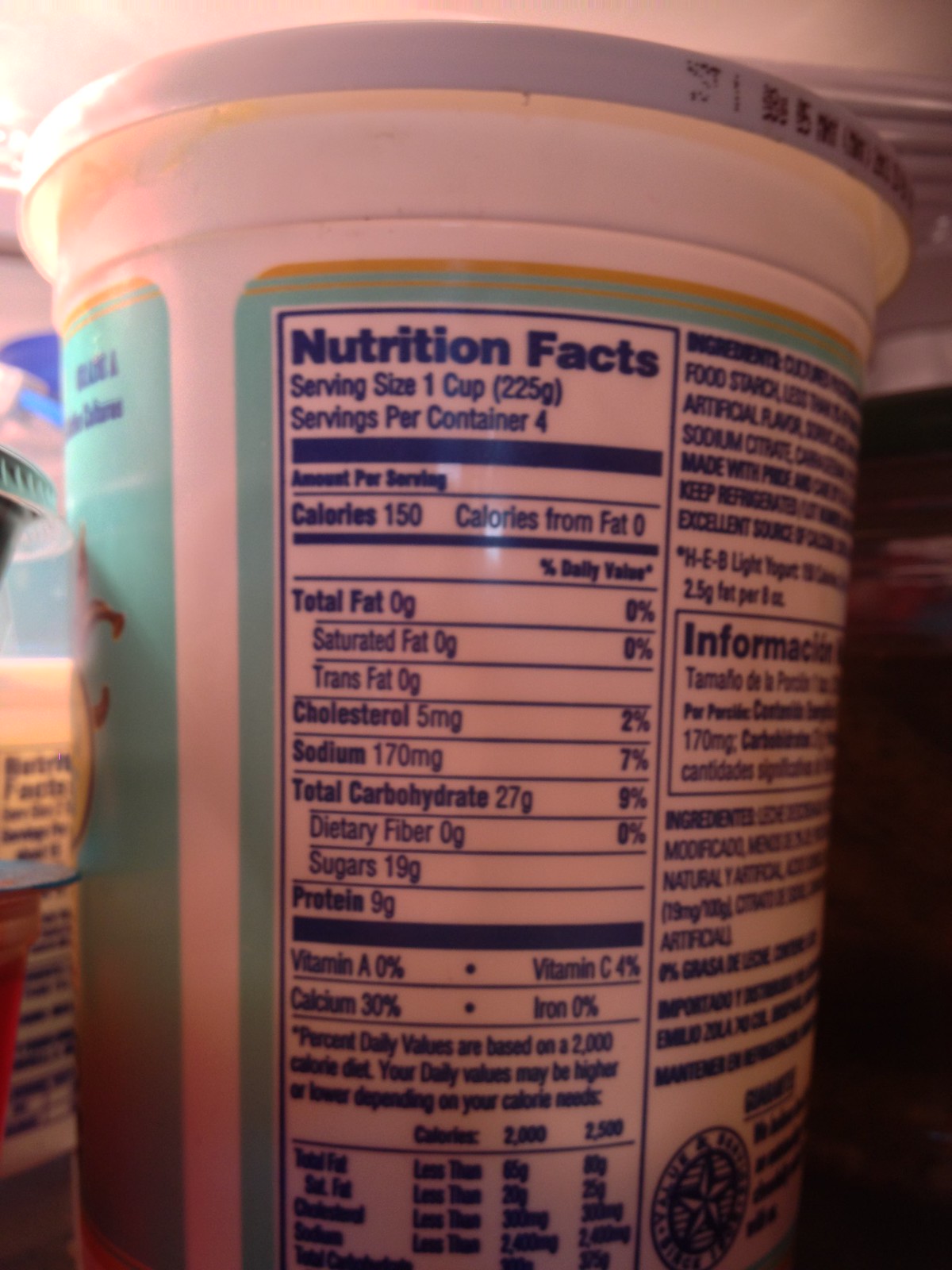This close-up photograph, taken inside a refrigerator, showcases the side of a large white plastic container, illuminated by a bright light shining from the upper left. The container features a white lid with black writing on the right, transitioning to a light teal background with a white strip down the side and an orange lining at the top. A teal border outlines the white section, which prominently displays the nutritional information in dark blue letters. The label details: "Nutritional Facts, serving size one cup (225 grams), servings per container: four." Below, it lists "Calories: 150, Calories from Fat: 0," followed by total fat (0 grams, 0%), cholesterol (5 grams, 2%), sodium (70 milligrams, 7%), total carbohydrates (27 grams, 9%), dietary fiber (0 grams, 0%), sugars (19 grams), and protein (9 grams). Unfortunately, the ingredients list on the right side is partially obscured as the label curves around the container. The overall appearance suggests the container might be holding yogurt, cottage cheese, sour cream, or ricotta, though the exact contents are not explicitly identified. The lower right corner of the image is dark, with some indistinct items visible in the background, emphasizing the tub as the primary focus.